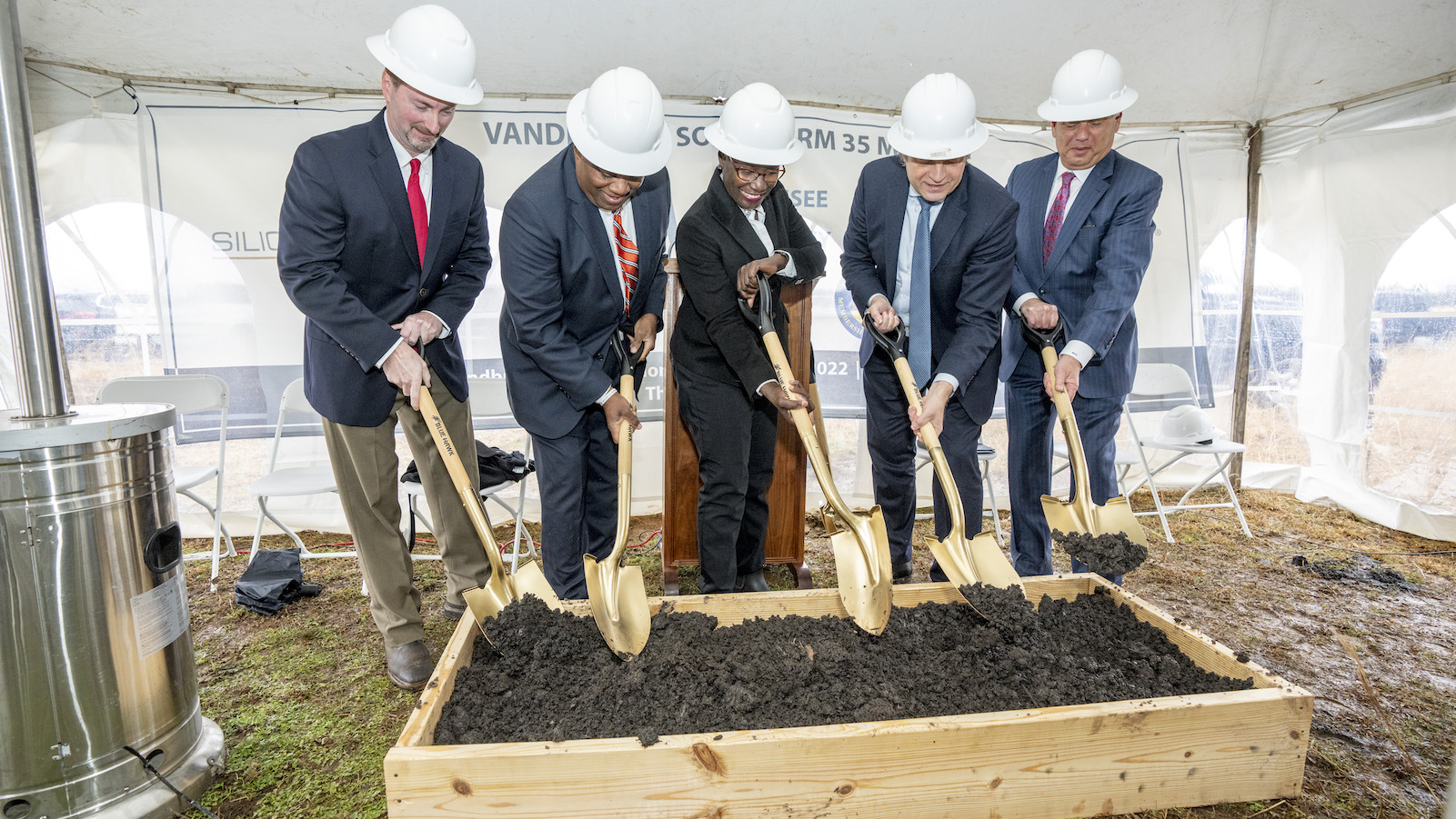A groundbreaking ceremony is captured in this photograph featuring a group of five individuals, consisting of four men and one woman, all dressed in formal attire. The men are wearing suits in shades of black and navy with ties, while the woman is attired in a white dress shirt. Each person is equipped with a gold shovel and a white hard hat, symbolizing the commencement of a new project. They are positioned under a large white tent, which has clear cutouts offering glimpses of the muddy grass and ground outside. White metal chairs can be seen arranged in the background, indicating an organized event setting. To the left side of the image, a large silver metal cylinder with an upward-extending pipe is visible, adding an industrial element to the scene. The group is actively digging into a blonde-colored wooden box filled with dirt, marking the ceremonial start of construction.